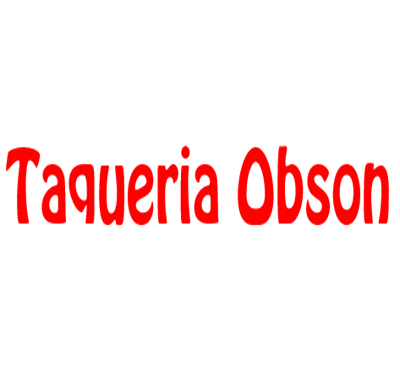The image features a striking, computer-generated graphic with bold red text on a solid white background. This text-only image displays the phrase "Taqueria OBSON" in a unique and somewhat whimsical, fat font. The letter "T" in "Taqueria" has a curved top, resembling an axe, while the "O" is distinctly egg-shaped. Notably, the "Q" in "Taqueria" lacks the typical tail, making it appear truncated. The text is split into "Taqueria" and "OBSON," with "Taqueria" in mixed case and "OBSON" in all capital letters. This captivating and oddly shaped lettering stands out crisply against the plain white backdrop, leaving a memorable visual impression.